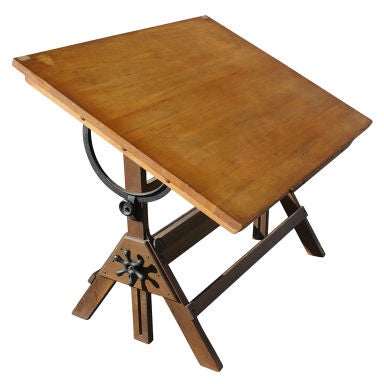The image captures a wooden drawing easel designed for architectural or engineering purposes, featuring a large, adjustable slanted surface ideal for blueprints or drawings. The main platform is a light brown wooden slab with a gradient of shades. Its angle can be modified using a half-round black lever positioned below, allowing for vertical to horizontal adjustments. The easel's structure sits atop a sturdy frame resembling a basic stool, consisting of triangularly arranged legs interconnected by horizontal wood beams, providing stability. Notable shadowing from an external light source accentuates the easel's form, highlighting key elements such as the adjustment lever and frame.